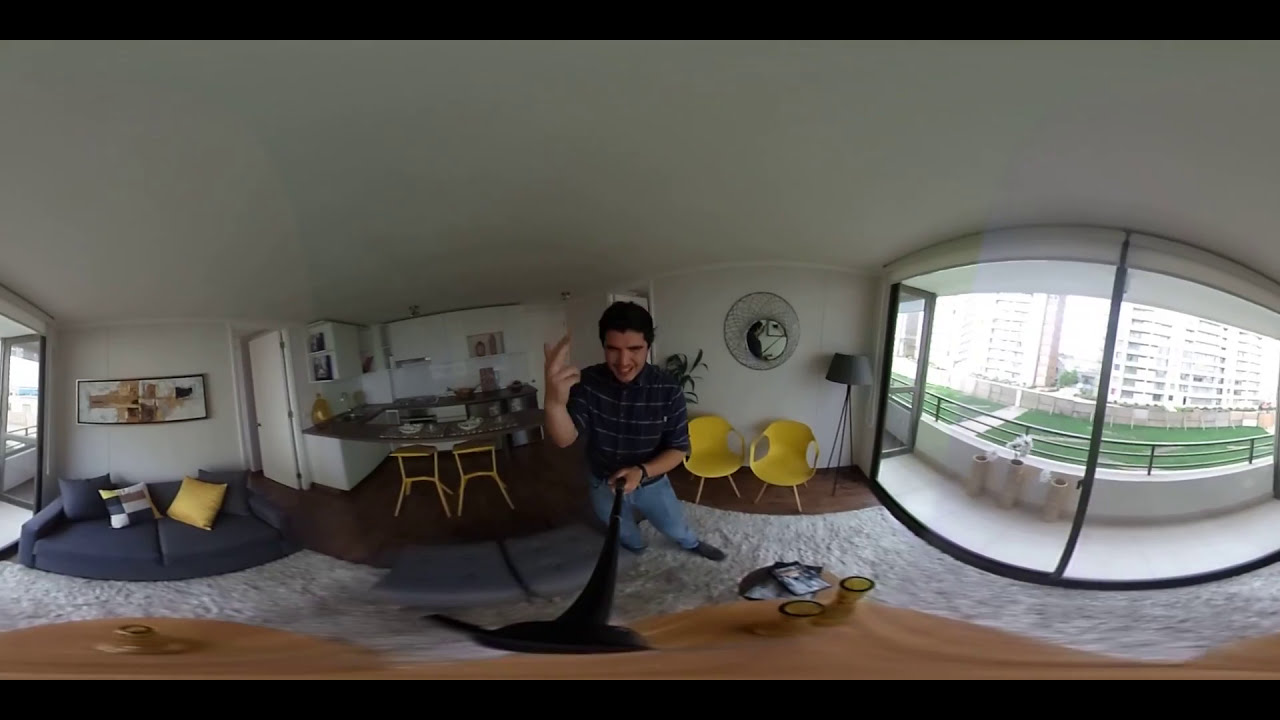A wide fisheye lens photo of an apartment several stories above ground level, bordered by thin black bars at the top and bottom. In the central section, a gentleman with short dark hair and dressed in a dark purple shirt with white lines and blue jeans is captured standing. He holds a black cloth in his left hand (on the right side of the image) and raises his right hand (on the left side of the image) while looking down. The scene around him is intricately detailed. 

To the left, a navy blue couch with two pillows, one yellow and one with a cubic design, sits against the wall adorned with abstract art. Below the couch, there is a white shag rug. 

Behind the man, there’s a kitchen area featuring white cabinetry and shelving, accompanied by a central dining table flanked by a couple of light yellow wood stools. In the foreground of the kitchen area, a light brown coffee cup is noticeable on the table. 

To the right of the gentleman, the living room extends towards an open window leading to a balcony. The balcony, enclosed by a gray metal railing, overlooks a grassy courtyard with surrounding multi-story white high-rise buildings visible in the background.

Highly detailed and filled with modern furnishings, the apartment conveys an inviting and lived-in atmosphere.